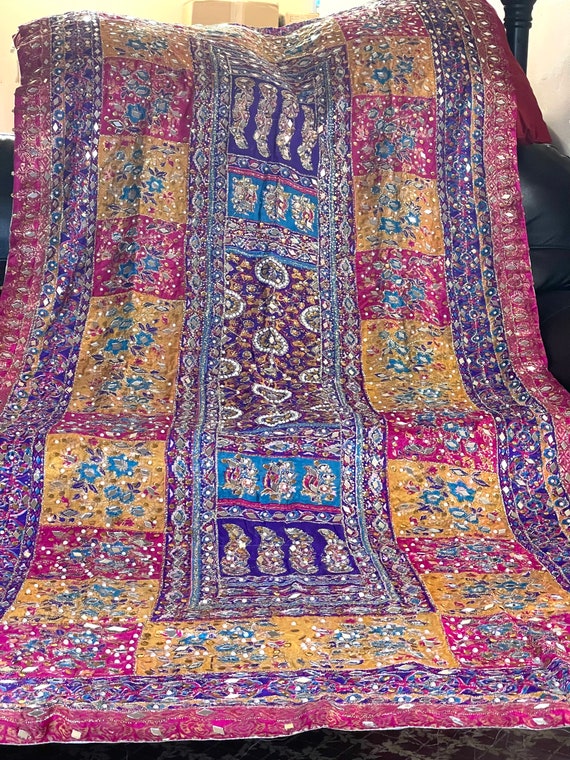A detailed photograph captures a handmade quilt that evokes a sense of Indian craftsmanship and design. The quilt is rich in a palette of colors including shades of red, burgundy, purple, white, yellow, blue, violet, rose, lavender, green, and turquoise. Dominated by a square pattern, the quilt features a central runner-style section flanked by square borders on the left and right. Each square patch showcases intricate paisley designs and floral motifs, some in pastel shades of yellow, blue, and turquoise. The outer borders of the quilt are deep purple, followed by an inner dark blue border that encloses a series of checkered squares in yellow and red. The central area is adorned with light blue and blue rectangles framed by intricate white drawings. Two solid color fabric edges outline the entire quilt, running continuously from bottom to top, left to right, and right to left, providing a polished finish to this vibrant and ornate creation.